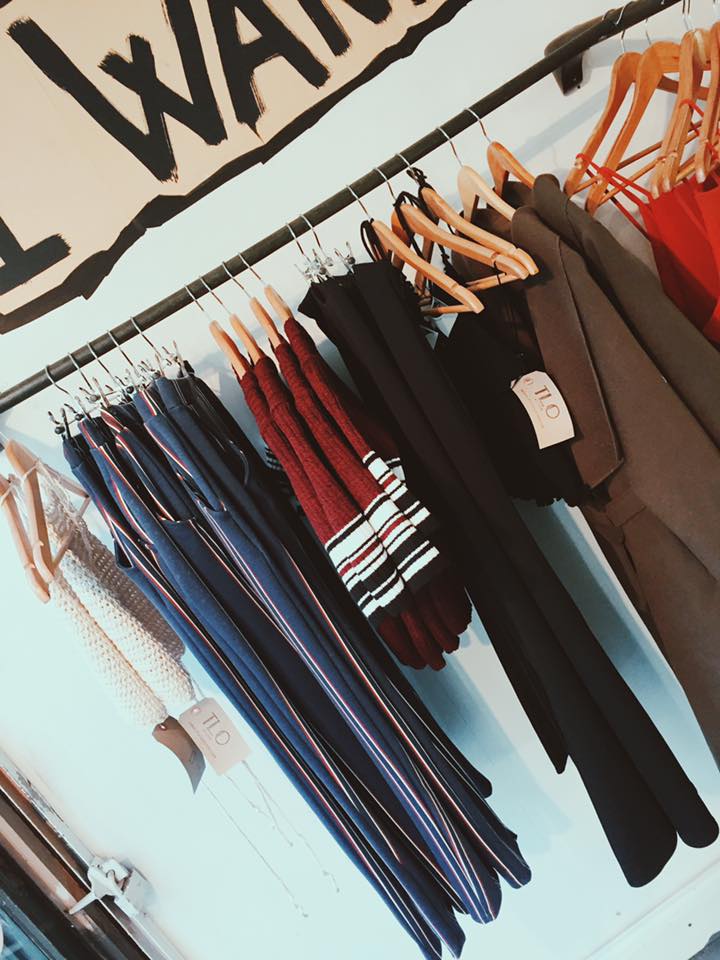A neatly organized clothing rack in a retail store is displayed against a powder blue wall. At the top left, there's a sign featuring black lettering on a cream background, outlining the section. Below the sign, a sleek black pole stretches across the display. From this pole, silver hangers suspend a variety of garments. 

On the far left, two oatmeal-colored skirts hang from brown wooden hangers. Next to the skirts, five pairs of trousers are lined up neatly. These trousers are predominantly blue with striking red stripes. Adjacent to the trousers, there are four tops exhibiting a vibrant mix of black, white, orange, and brown stripes, gradually transitioning to a brown hue at the bottom.

Following these tops, two pairs of black pants are displayed with an indistinguishable black item sandwiched in between. To the right of the black clothing items, two elegant brown coats are hung. Lastly, the display concludes with two or three red sleeveless blouses. Most of the garments are suspended from brown wooden hangers, while the pants are secured with metal clips, providing a uniform and tidy presentation.